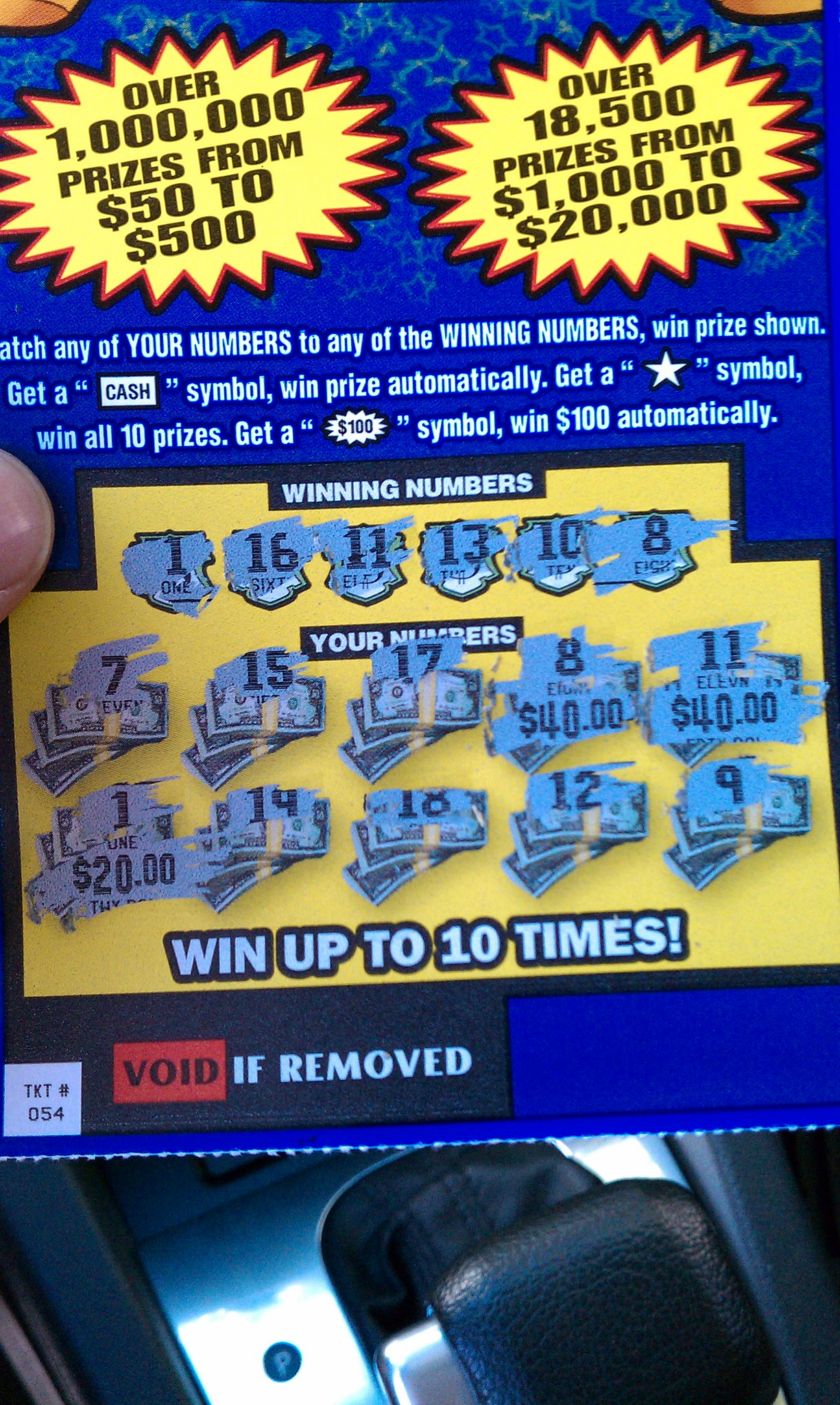The image is of a blue scratch-off lottery ticket, which appears slightly torn at the bottom and held up by the owner's left hand. The ticket displays a detailed blue and yellow design featuring two yellow starburst sections at the top. The left starburst announces "Over 1 million prizes from $50 to $500," while the one on the right states "Over 18,500 prizes from $1,000 to $20,000." The instructions "Match any of your numbers to any of the winning numbers, win prize shown. Get a cash symbol, win prize automatically. Get a star symbol, win all 10 prizes. Get a $100 symbol, win $100 automatically," are prominently printed. 

The winning numbers listed at the top of the ticket are 1, 16, 11, 13, 10, and 8, while the player's numbers are 7, 15, 17, 8, 11, 1, 14, 18, 12, and 9. The player has matched the number 1 three times for $20 each, the number 8 twice for $40 each, and the number 11 once for $40, totaling $100 in winnings. The lottery ticket also has a notice at the very bottom stating "Void if removed." The picture appears to be taken inside a car, with part of the gear shift visible below the ticket, and the owner's thumb can be seen holding the edge of the ticket on the left.